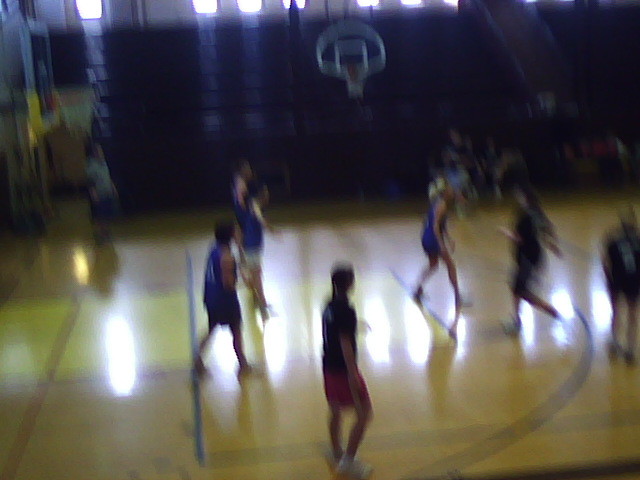This is a very blurry image of a women's basketball game in progress, likely at the high school level. The photograph captures several players on the court, most of whom appear to be in motion, adding to the blurriness. The teams are distinguishable by their uniforms, with one team in blue and purple jerseys and the other in darker tops, possibly black. The court is a polished blonde wood color, marked with standard basketball stripes. Two basketball goals are visible; one prominently to the left, which features an orange rim, a white net, and an orange-painted base. Another goal can be seen hanging in the background. The stands are sparsely populated with a few scattered individuals, suggesting this could be a practice session rather than a formal game. The venue has windows at the top, allowing light to reflect onto the court, further contributing to the blurry nature of the image.